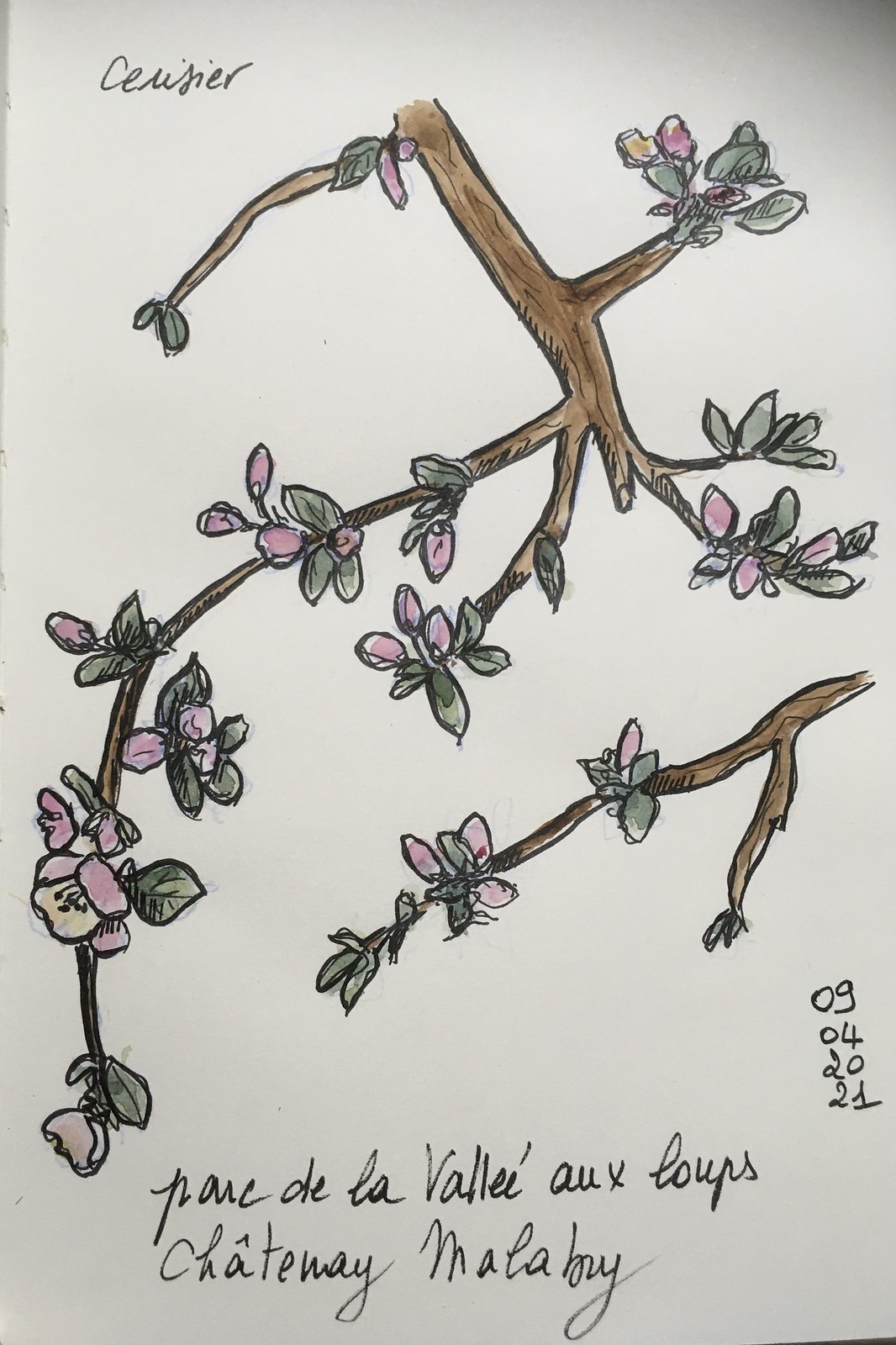In this rectangular image, we see a meticulously hand-sketched and colored artwork. In the upper left corner, the word "CEUNER" is prominently written, possibly indicating a name or title in a different language. Below this, amidst a beautifully intricate arrangement of flowers on branches, there is text in French that reads "Parc de la Vallée-au-Loup, Chatemag Malaboy." A date, "09-04-2021," is inscribed in black ink, adding a temporal reference to the scene.

The drawing features brown branches that extend from the upper left and lower right corners, creating a dynamic sense of movement. Delicate pink flowers, each adorned with green leaves, are scattered throughout the branches. The artist has used a combination of black thin marker to outline the elements, and colored pencils or possibly light paint for filling in the colors. The contrast between the soft hues of the flowers and the bold outlines enhances the overall visual appeal, showcasing the artist's skill in both drawing and coloring techniques.